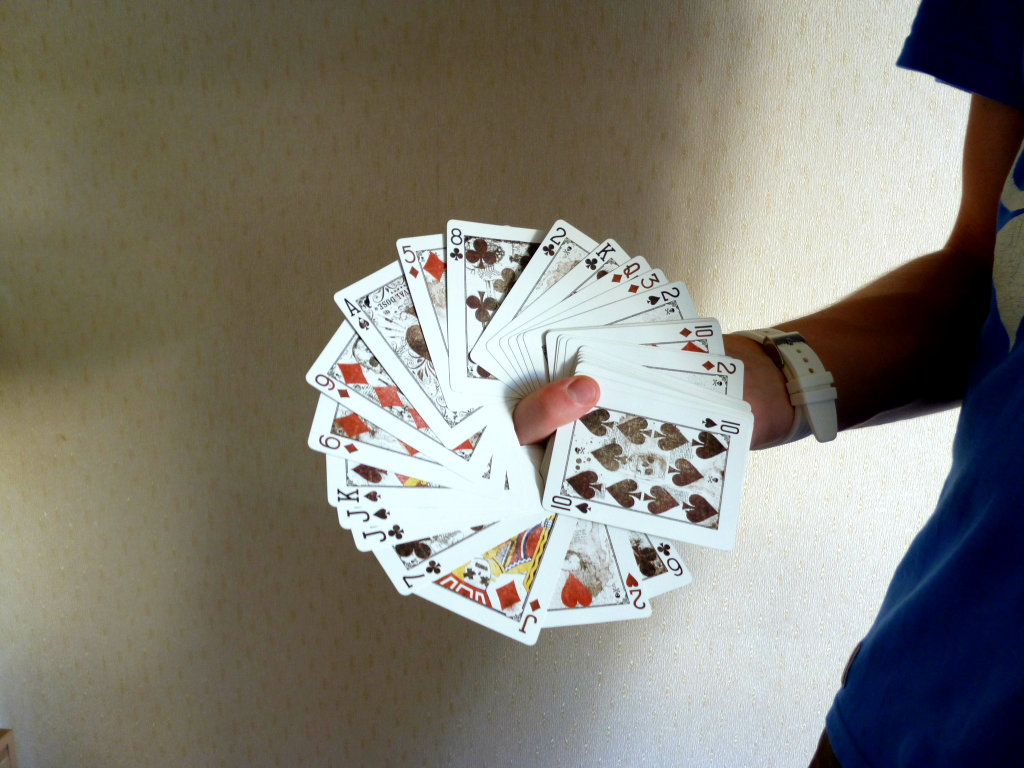A dynamic photograph captures a possibly Caucasian individual wearing a blue, floral short-sleeved shirt with white lettering. The person’s arm is bent, showcasing a white watch with a visible band. They are turned sideways against a white wall speckled with small dots, adding texture to the background. 

In the center of the image, the individual's thumb can be seen, around which a circular spread of playing cards floats. The spread includes a variety of cards with only their indices and suit symbols visible, creating a mesmerizing pattern. Prominent among the cards, the ten of spades is fully displayed, adorned with black spade symbols. Other visible cards in the spread include the two of diamonds, ten of diamonds, two of spades, three of diamonds, queen of diamonds, king of clubs, two of clubs, eight of clubs, five of diamonds, eight of spades, nine of diamonds, six of diamonds, king of spades, jack of spades, jack of clubs, seven of clubs, jack of diamonds, and six of clubs. Each card features a clean white background, contributing to the clarity and coherence of the circular display. The image beautifully blends elements of magic and precision, highlighting the dexterity and skill of the individual.